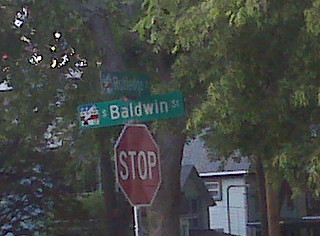The image features a bustling urban street scene. At the forefront, there is a prominent red stop sign with white lettering. Surrounding the stop sign are green street signs, with one clearly displaying "Baldwin Street" in the center. To the left of the main sign, there's a small square sign whose details are unclear, and at the top, another sign is partially visible with unreadable text.

On the right side of the image, there stands a tall tree with lush green leaves, while another tree is positioned more centrally. These trees frame the scene with their verdant foliage extending around the top edges of the image.

In the background, a residential building can be seen. The building features an open gate, a distinctive gray sloped roof, and siding made of white wood. Additionally, blue slopes add contrast to the structure, and the sky above is overcast, casting a white hue across the scene.